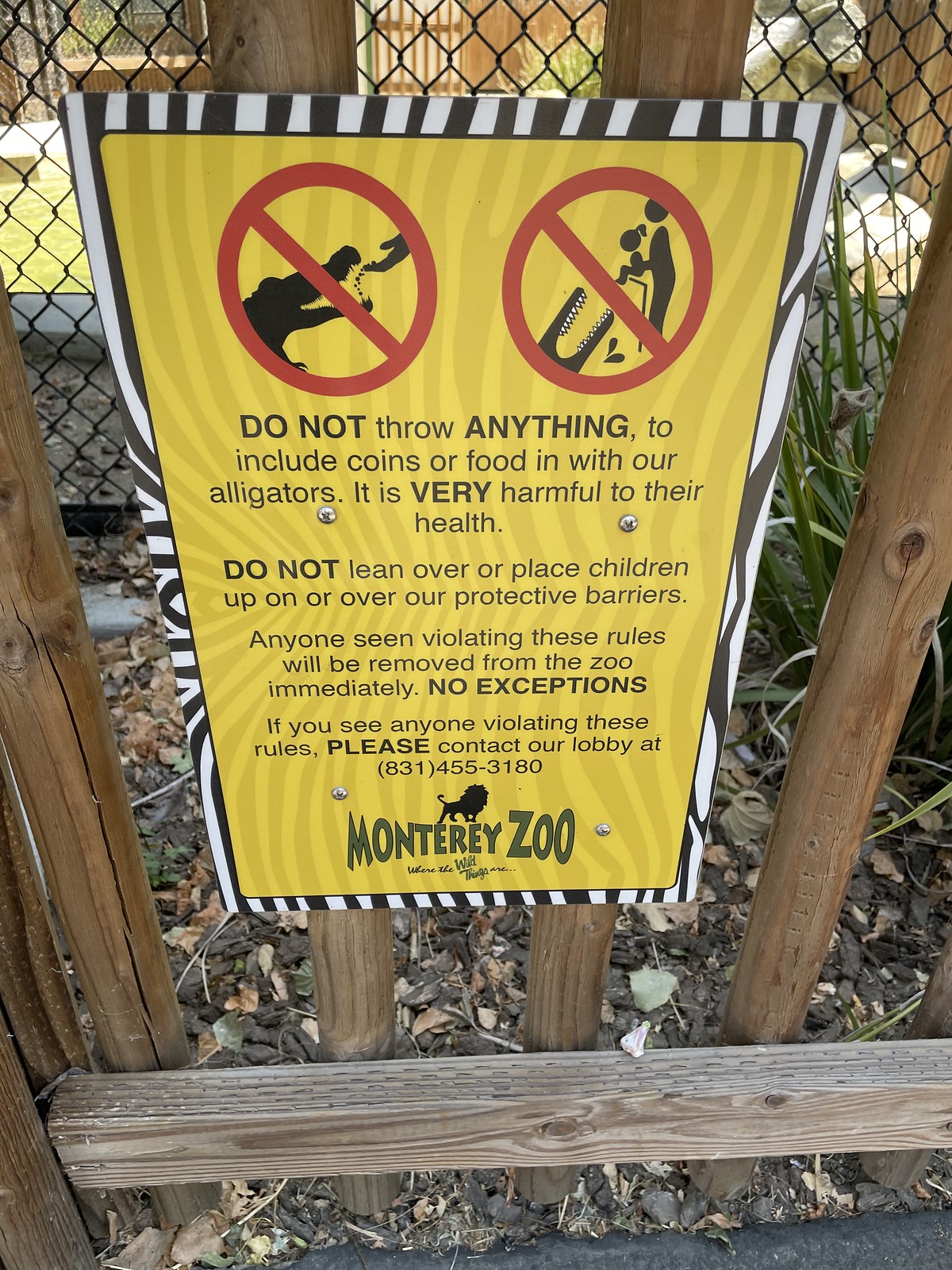The image depicts a cautionary sign mounted on a wooden fence at the Monterey Zoo, with a chain-link fence and foliage visible in the background. The sign features two prominent "do not" icons—red symbols with a line through them—indicating prohibited actions. One icon shows a person attempting to feed an alligator, while the other depicts a person lifting a child over a fence. Beneath these images, the text reads: "Do not throw anything, including coins or food, in with our alligators. It is very harmful to their health. Do not lean over or place children upon or over our protective barriers. Anyone seen violating these rules will be removed from the zoo immediately. No exceptions. If you see anyone violating these rules, please contact our lobby at 831-455-3180." The sign emphasizes strict adherence to these regulations for the safety of both visitors and animals. At the bottom of the sign, the Monterey Zoo logo is displayed, featuring a silhouette of a lion.